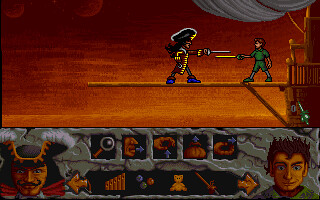The image is a small, pixelated screenshot from an old video game, depicting a dramatic sword fight. The scene, seen from a pirate ship's viewpoint, features a reddish-brown sky and a wooden plank extending out from the ship. On this plank, two iconic characters confront each other: Peter Pan, dressed in green with shorts and top, faces away from the ship with a gold sword. Opposite him is Captain Hook, adorned in classic pirate regalia including a red coat, blue shoes, and a prominent captain's hat, wielding a silver sword. Their swords are crossed horizontally as they duel. Above them, the ship's sails are faintly visible, contributing to the nautical atmosphere. The bottom third of the screen displays a game menu with close-up images of Captain Hook on the left and Peter Pan on the right, along with various icons, including a magnifying glass, indicating interactive elements or gameplay options.